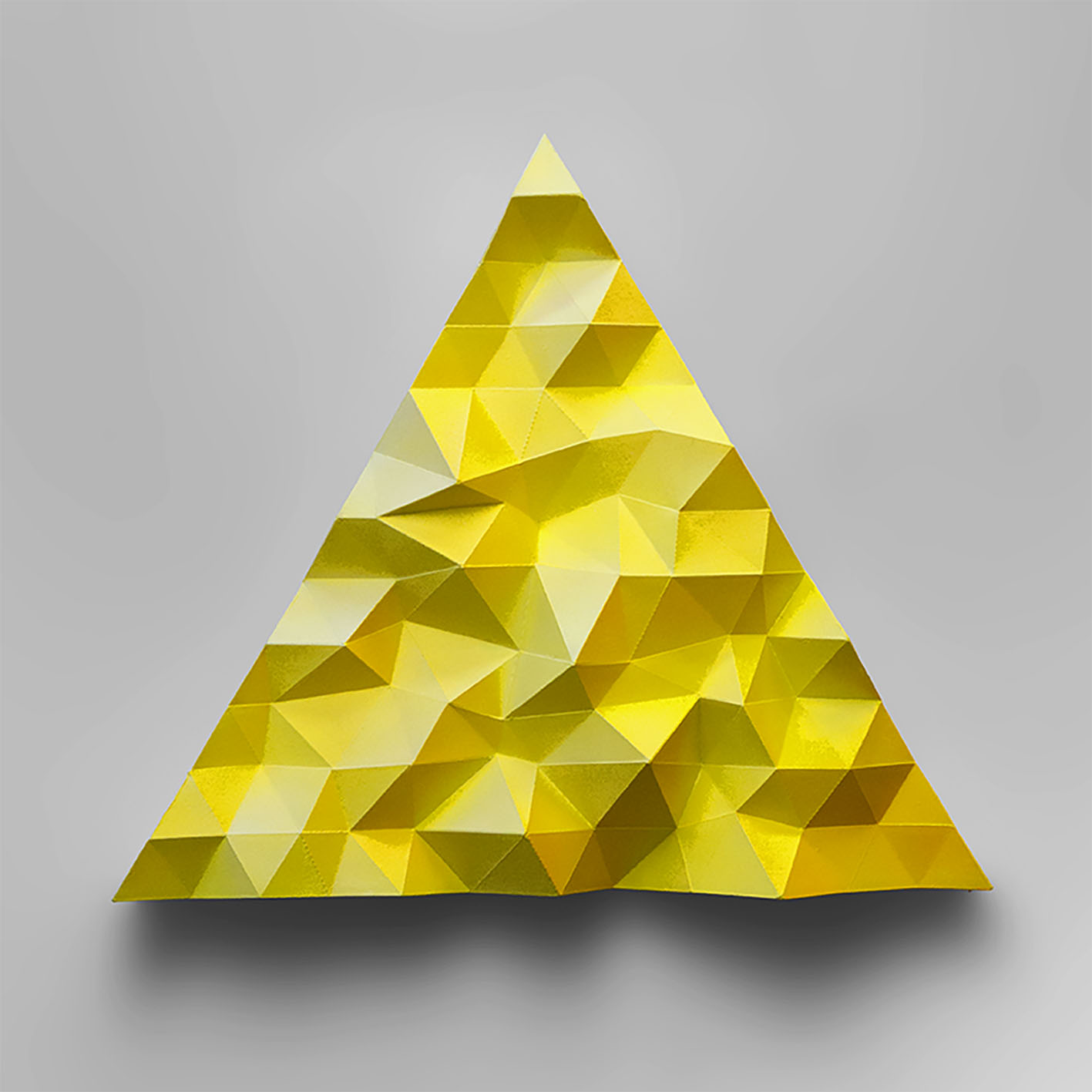This is a detailed color photograph of a meticulously crafted origami sculpture placed on a light gray surface. The centerpiece of the image is a yellow triangular paper with the base at the bottom and the point at the top. The paper is artistically folded into numerous pyramid-like shapes that create a textured surface, featuring depressions and elevations that give an impression of a multi-faceted structure. The intricate folds and protrusions result in sections that exhibit a gradient of colors from light yellow and cream to dark yellow and brown, depending on the angle and lighting. The lighting, which comes from the top, enhances the three-dimensional effect and casts a shadow at the bottom, further highlighting the detailed craftsmanship of the origami piece.